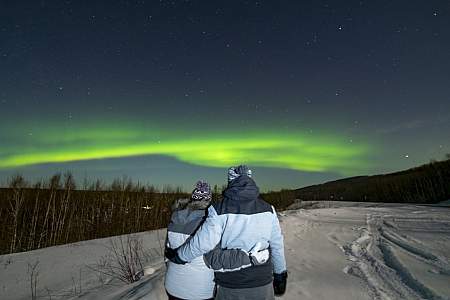In the evening under a star-speckled, dark blue night sky, a couple stands in a vast, snow-covered field surrounded by a dense forest of barren trees and scattered shrubs. Dressed in full winter gear, including blue jackets, mittens, and toboggans, they embrace each other, gazing at the mesmerizing neon green and yellow hues of the northern lights stretching across the horizon. The woman's jacket is adorned with a fur hood. Car tracks are visible in the snow to their right, adding a subtle, human touch to the serene and expansive natural landscape.